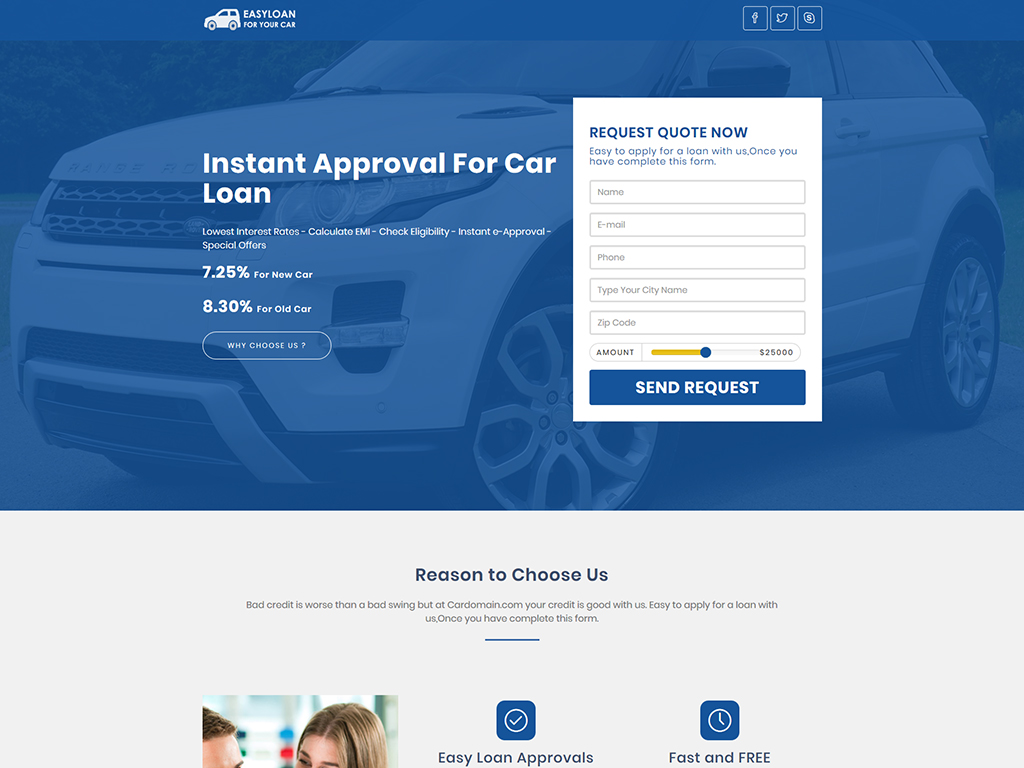Screenshot of the "Easy Loan for Your Car" Website:

The webpage features a sleek design with a blue header at the top displaying the company name on the left and icons for Facebook, Twitter, and Snapchat on the right. Adjacent to the title is an image of a white card, adding a visual touch.

Below the header, the page is divided into two sections. The left section, predominantly blue, showcases a white SUV with a header reading "Instant Approval for Your Car Loan." This section mentions loan terms: 7.25% for a new car and 8.30% for an old car, highlighting their competitive rates. A prominent white button labeled "Choose Us" is easily accessible for users.

On the right side, there's a floating white box with blue text that invites users to "Request a Quote Now." It includes fields for entering a name, email, phone number, city, and zip code. Additionally, there’s a sliding bar allowing users to select a loan amount up to $25,000. Below this slider is a blue button labeled "Send Request."

The lower portion of the webpage transitions to a gray background, centered with the title "Reasons to Choose Us." Despite some text being cut off in a picture insert, there are clearly two icons: one showing an "Easy Approval" with a blue checkmark, and another indicating "Fast and Free.” 

This well-organized layout ensures a user-friendly experience while clearly outlining the services and benefits of opting for an Easy Loan for your car.